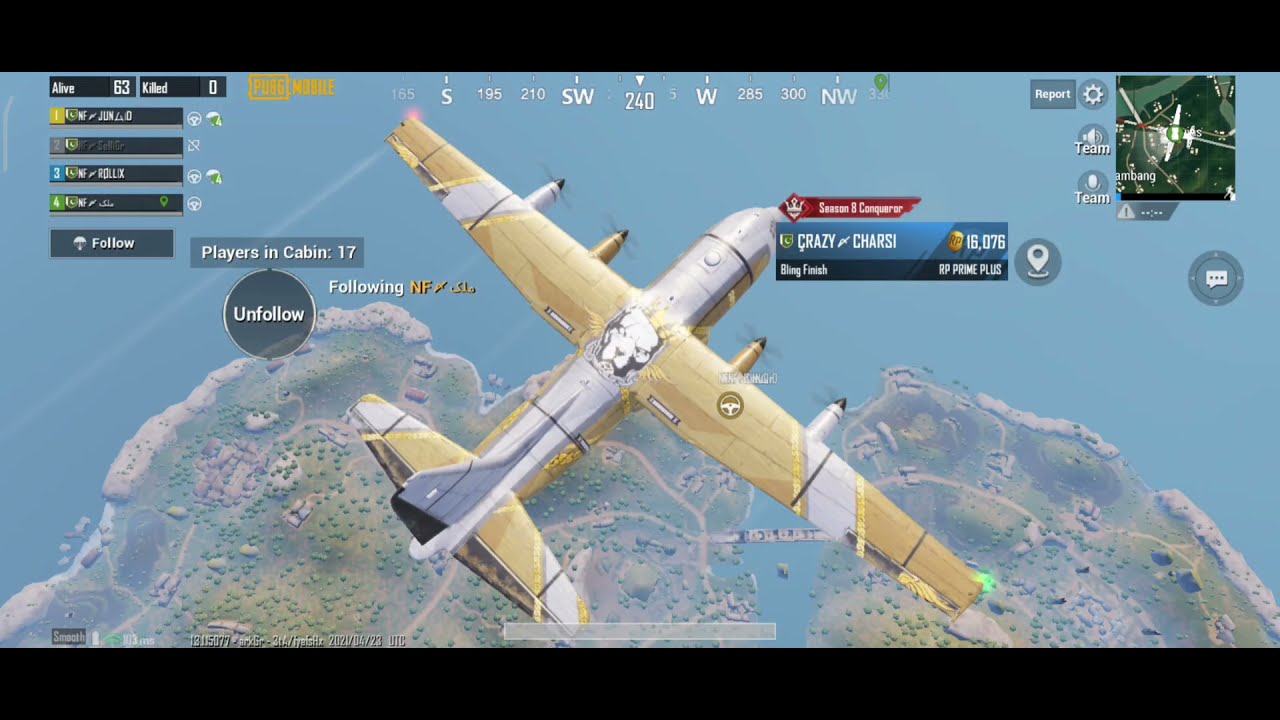The image is a highly detailed screenshot from a video game, showcasing an overhead view of an animated fighter plane flying over a blue ocean and islands. The plane features a silver fuselage, gold wings adorned with diagonal gray stripes, and a white tail with a single black stripe. Its center bears a lion face design. Each wing has two motors—one white and one gold. Situated prominently in the middle of the plane, a banner reads "Crazy Kasi," with "Season 8 Conqueror" above it, followed by "Binge Finish," the score "16,076," and "RP Prime Plus" below. The top of the screen displays a navigation gauge with compass headings—S for South at 195°, 210°, SW, 240°, W, 285°, 300°, and NW. The upper right corner features a green map location square labeled "Report," alongside gear and speaker icons, with "Team" under the speaker icon and microphone icon. The upper left corner includes statistical bar graphs labeled 1, 2, 3, and 4, and a smaller banner saying "Follow." Above that, two more gray banners indicate "Above, Alive 63" and "Kill to Zero." A black strip runs across the top and bottom of the screen, filling empty space.